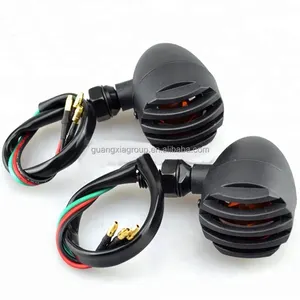The image features two identical black electrical devices positioned side-by-side against a plain white background. Each device is cone-shaped, tapering down to a slightly wider base, and topped with a plastic panel resembling a vent or fan guard, consisting of black slats with spaces in between, suggesting it could function like an air conditioning vent. From the base of each cone, a thick black cable extends out, supplemented by additional thinner wires wrapped in black electrical tape. Among these wires, a red and a green cable are prominently coiled around the main black cable, and all converging cables terminate in gold-colored connectors. The devices appear to be labeled with the brand "Guangxia group sn.alababa.com." The intricate details of the wiring and the fan-like component suggest these are electrically functional, possibly serving a mechanical or automotive purpose.